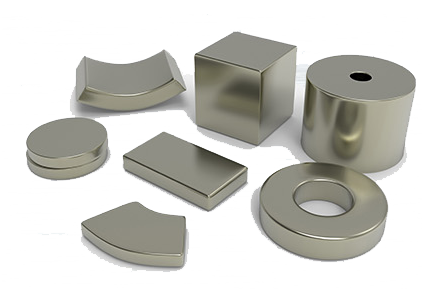The image showcases seven distinct three-dimensional, metallic shapes arranged on a white surface. These shiny, reflective objects include a variety of forms: at the top left, a 3D arc piece, followed by a cube, and a cylinder with a hole in the center. In the middle row, there are two stacked circular pieces, a rectangle reminiscent of a silver bullion bar, and a donut-shaped ring. At the bottom, there is another arc piece. Each shape is silver-colored, giving the appearance of polished metal.